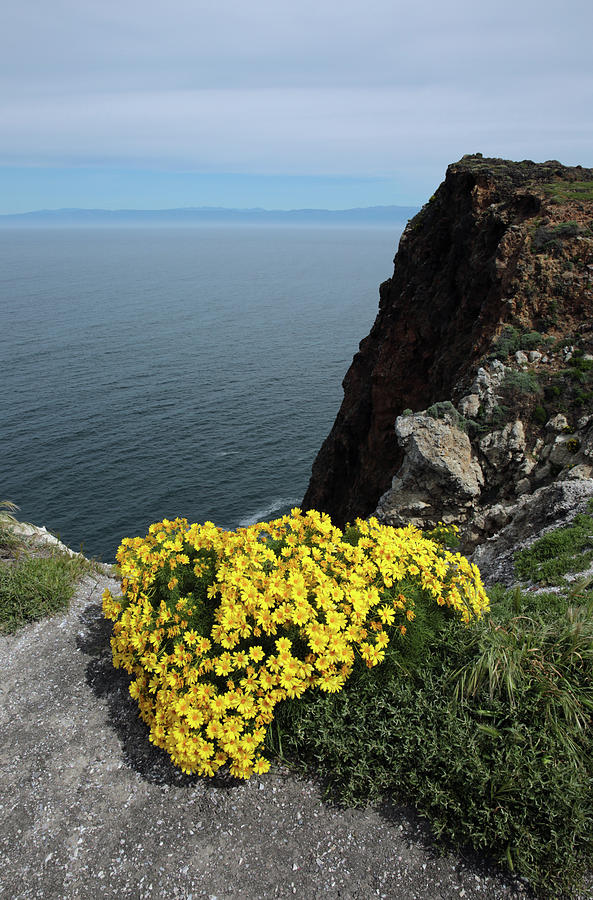This captivating photograph captures the stunning view from a cliffside, presenting a harmonious blend of earth, sky, and sea. In the foreground, the edge of the cliff is prominently featured with gray stone rock and a patch of vibrant yellow wildflowers in full bloom next to a tuft of green grass. The cliff itself shows a gradient of colors—the darker, mossy brown upper sections transitioning to the grayish, sun-baked lower areas. To the right, another cliff edge rises higher towards the sky.

Beyond the cliff, the calm, clear waters stretch out under a sky that oscillates between cloudy with patches of blue. The expansive body of water, potentially an ocean or a large lake, reflects the serene sky, creating an almost mirror-like effect. In the distance, the hint of another landmass or mountain range can be seen, casting a shadow across the water, adding depth to the scene. The photograph captures the serene beauty of nature, combining the rugged cliffside, the tranquil ocean, and the expansive, partly cloudy sky. Overall, it portrays an idyllic, peaceful day with a perfect blend of natural elements.